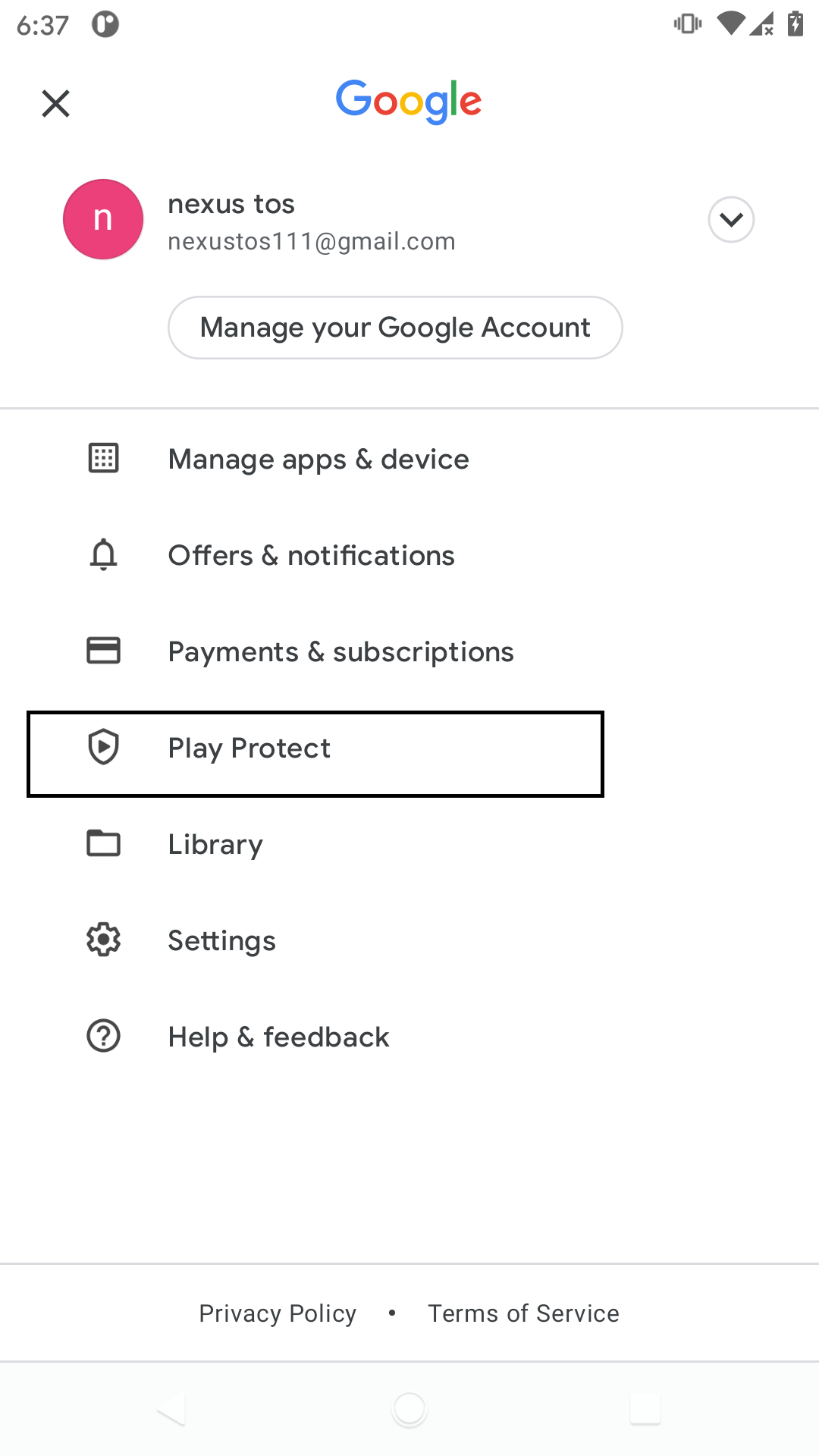The image depicts the detailed interface of managing Google accounts. At the top left, the number "37" is visible, likely indicating a notification count. A vibration icon follows, indicating that the device is on vibrate mode. The Wi-Fi icon shows full signal strength, while the network symbol temporarily displays "no signal." Despite this, the battery indicator shows it is almost full.

At the center, the Google logo is prominently displayed, featuring the iconic multicolored letters "G-O-O-G-L-E." Below the logo, there's a pink circle with the letter "N" in the middle, next to text that reads "NEXUSTOS111@gmail.com," accompanied by a dropdown arrow.

Directly below, an oval button reads "Manage your Google Account," separated by a divider line from the next section. This next section includes "Manage Apps and Device," represented by an icon with 9 dots arranged in a square. Adjacent to these, there's a bell icon for notifications, followed by the "Offers and Educations" section.

Further sections include:
- An icon resembling a credit card for "Payments and Subscriptions."
- A highlighted shield with a play button inside, representing the selected section.
- An embedded folder icon, a window icon, and a gear icon, likely denoting additional settings or sections.
- A "Friends" section, followed by a circle with a question mark inside indicating "Help and Feedback."

The bottom portion of the interface features a divider line, followed by links to "Privacy Policy," denoted with a separating dot, and "Terms of Service," ending with another divider line.

This comprehensive layout is indicative of the settings page for managing various aspects of Google accounts.